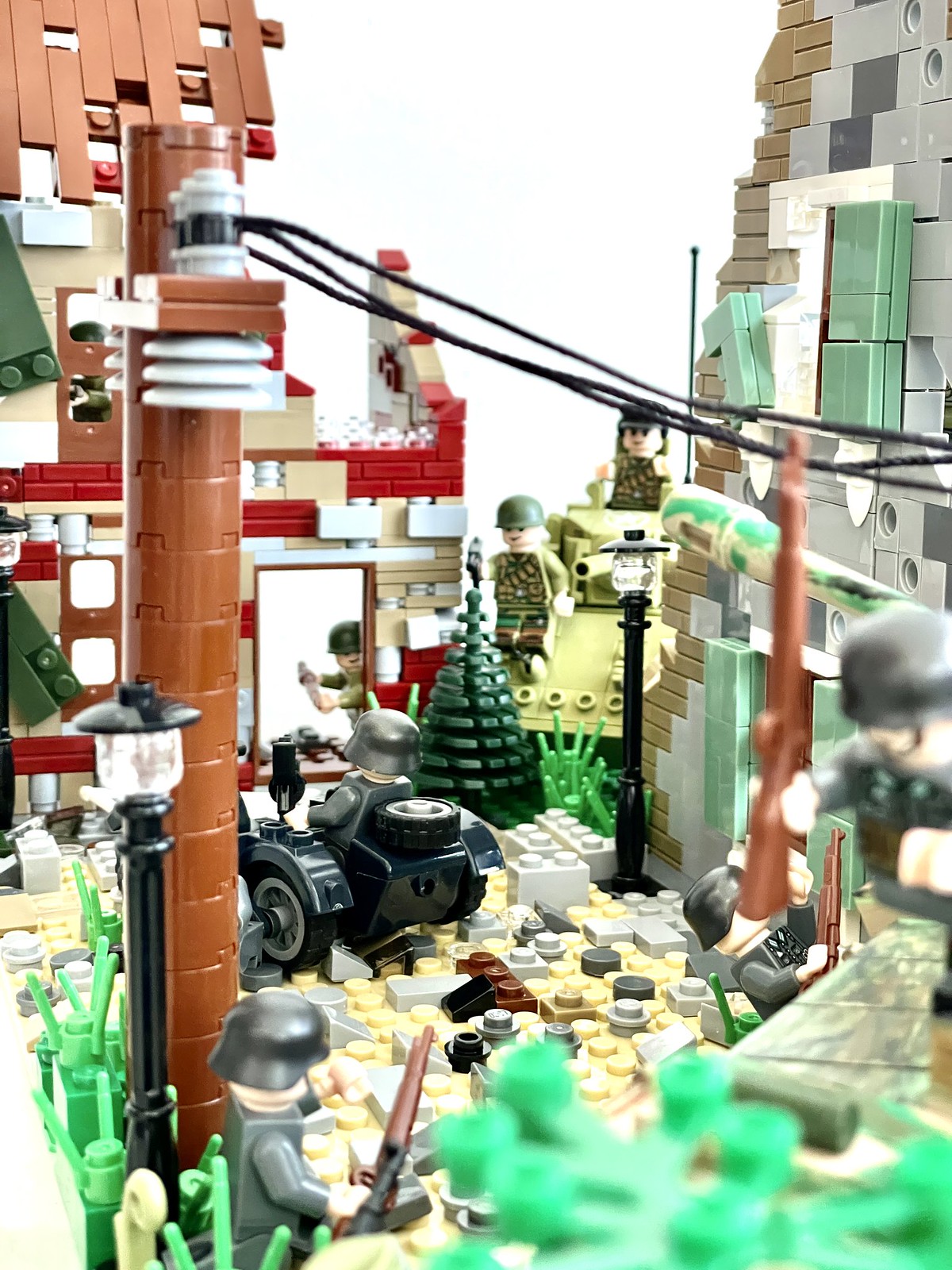The photograph captures an intricate Lego construction designed to resemble a battlefield scene. Centered in the image, there are remnants of two buildings. The first, made with light tan and red bricks, has a slanted brown roof, a broken-open side revealing its interior, and a door at the bottom. Nearby, a Lego figure dressed in a green uniform and helmet leans outward, holding a bomb as if preparing to throw it. Adjacent to this building is a small Lego trike or Jeep with a figure in a grayish uniform seated inside.

To the left, a long brown wooden telephone pole extends across the scene horizontally, with black shoelace-like wires mimicking power lines. An ornate dark green evergreen tree adds detail to the setting. Scattered around the scene are army men, including one in a gray uniform with a rifle in the lower left corner and another in gray with a brown rifle positioned just above the lower right corner. Near the right-hand side, the gray remnants of another building appear, also broken open. From this side extends a long tank barrel, while a green tank advances from the center-right, manned by green-uniformed soldiers—one in front and one inside its back.

The ground below is variegated to emulate rock or gravel, with patches of black, dark gray, dark brown, light gray, and yellow. A streetlight stands tall amidst the scene, alongside a strip of barbed wire that runs along the side of the street, adding to the wartime atmosphere. The sky above is dull and featureless, blending into the top center of the frame, which is whited out, enhancing the focus on the chaotic ground action below.